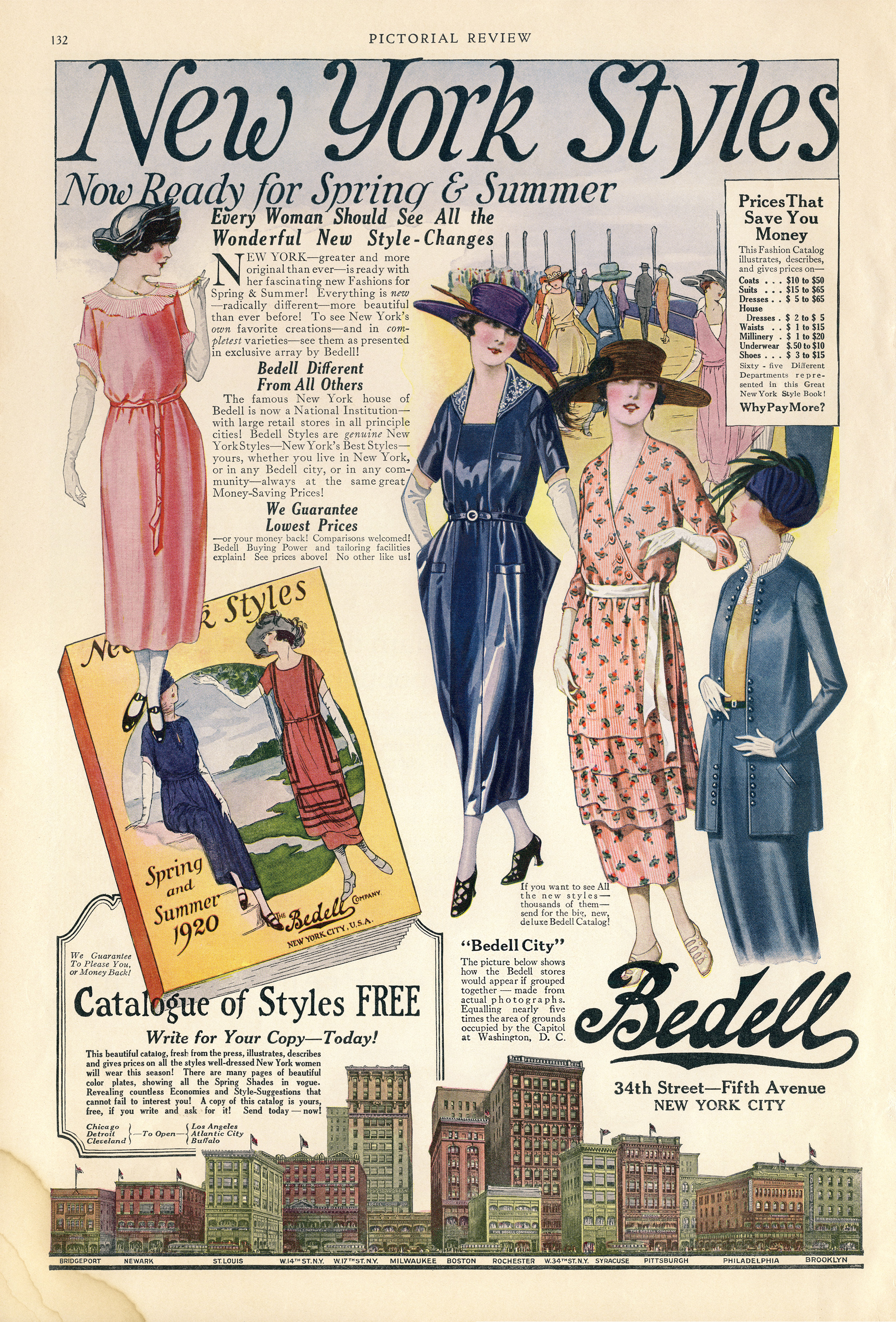This is a vintage fashion catalogue advertisement, sepia-toned and titled "New York Styles Now Ready for Spring and Summer," featured prominently at the center top beneath a smaller heading, "Pictorial Review." The catalogue proudly proclaims, “Every woman should see all the wonderful new style changes. New York, greater and more original than ever, is ready with her fascinating new fashions for spring and summer. Everything is radically different, more beautiful than ever before.” 

The advertisement showcases animated paintings of women dressed in various stylish outfits and hats. On the left, below the headline, a woman is adorned in a red dress with short sleeves and a black hat decorated with flowers on the rim. In the middle of the illustration, three women are portrayed; the central figure wears a tall black hat with a white rim, paired with a shiny blue dress cinched by a black belt. To her right, a woman is seen in an orange dress with a white belt and floral pattern. Next to her, on the far right, stands a woman in a blue shirt and pants, matched with a yellow shirt underneath and accessorized with a hat featuring black feathers. 

The background art depicts a cityscape of brown and green buildings, reinforcing the New York ambiance. Additional text promotes BEDL, a paramount New York fashion house, offering their catalogue of styles for free. It highlights BEDL's vast range of fashion items, from suits to millinery, available at guaranteed lowest prices, urging readers to write for their copy today. The ad concludes with the BEDL brand name and addresses, including their main store at 34th Street, Fifth Avenue, New York City.